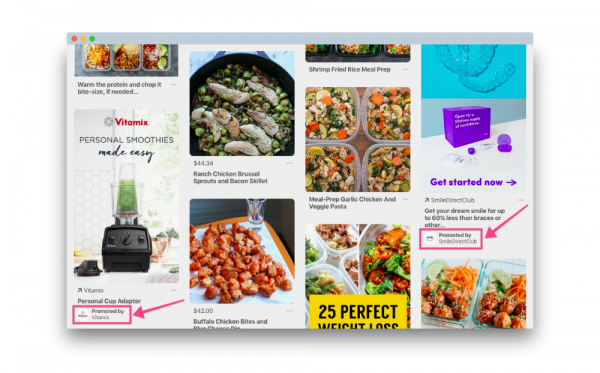The screenshot showcases a webpage with various images and advertisements, organized as follows:

1. **Header Icons**: At the top, there are matte red, yellow, and green dots within a gray rectangle, indicating the window controls.
  
2. **Meal Instructions and Photos**:
   - **First Image**: A meal comprised of three separate compartments, accompanied by the instruction: "Warm the protein and chop it bite-size if needed."
   - **Second Image**: A large frying pan filled with chicken and Brussels sprouts, labeled "4433. Ranch Chicken, Brussels Sprouts, and Bacon Skillet."
   - **Third Image**: Text reading "Shrimp Fried Rice Meal Prep," with only a portion of the corresponding image visible.
   - **Fourth Image**: "Meal Prep Garlic and Veggie Pasta" displayed across four plastic containers.

3. **Advertisements**:
   - **Bottom Left Corner**: A Vitamix ad highlighting "Personal Smoothies Made Easy with 28 vitamins and a Personal Cup Adapter," presented by Vitamix.
   - **Moving Right**: An image of food on a square white dish with an orange border, captioned "Buffalo Chicken Bites and Blue Cheese Dip" priced at $42.
   - **Next Ad**: A collection of foods within plastic containers, partially labeled "25 Perfect Weight Loss" (with the rest cut off).
   - **Far Right**: A prominent ad for Smile Direct Club, featuring a large aqua-colored rectangle with an illustration of a purple box and related items. The text reads: "Get started now," followed by "Smile Club Direct. Get your dream smile for up to 60% less than braces or other. Presented by Smile Direct Club."

4. **Cut-off Images**: At the very bottom right, there are partially visible images of two different types of meals.